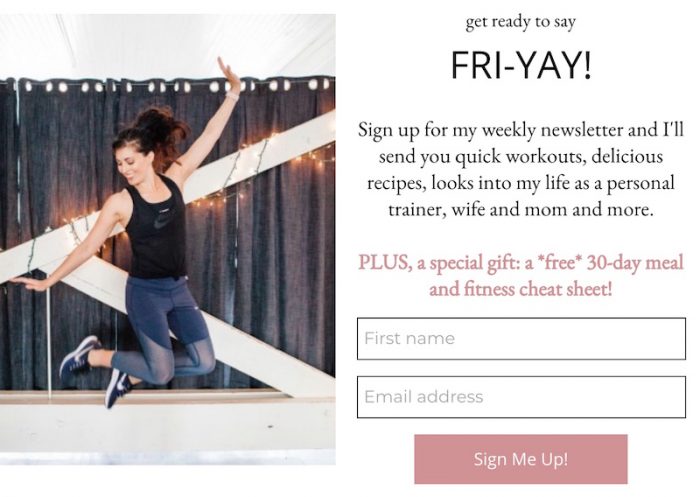This is a screenshot from an online advertisement featuring a dynamic scene of a woman mid-dance. She is wearing a black shirt paired with tight, jean-like leggings and blue and white shoes, captured in mid-air with her feet off the ground and arms spread wide. She performs against a backdrop of a blue curtain adorned with lights, suggesting a stage setting. 

To the right, the ad text energetically invites viewers with the headline: "Get ready to say FRIYAY!" Below this, the advertisement encourages sign-ups for a weekly newsletter, offering quick workouts, delicious recipes, glimpses into the life of a personal trainer, wife, and mom, and more. Additionally, in pink lettering, the ad entices with the promise of a special gift: a free 30-day meal and fitness cheat sheet. Beneath this offer are two text fields - one for the first name and the other for an email address. At the bottom, a prominent pink button with the text "SIGN ME UP" beckons potential subscribers.